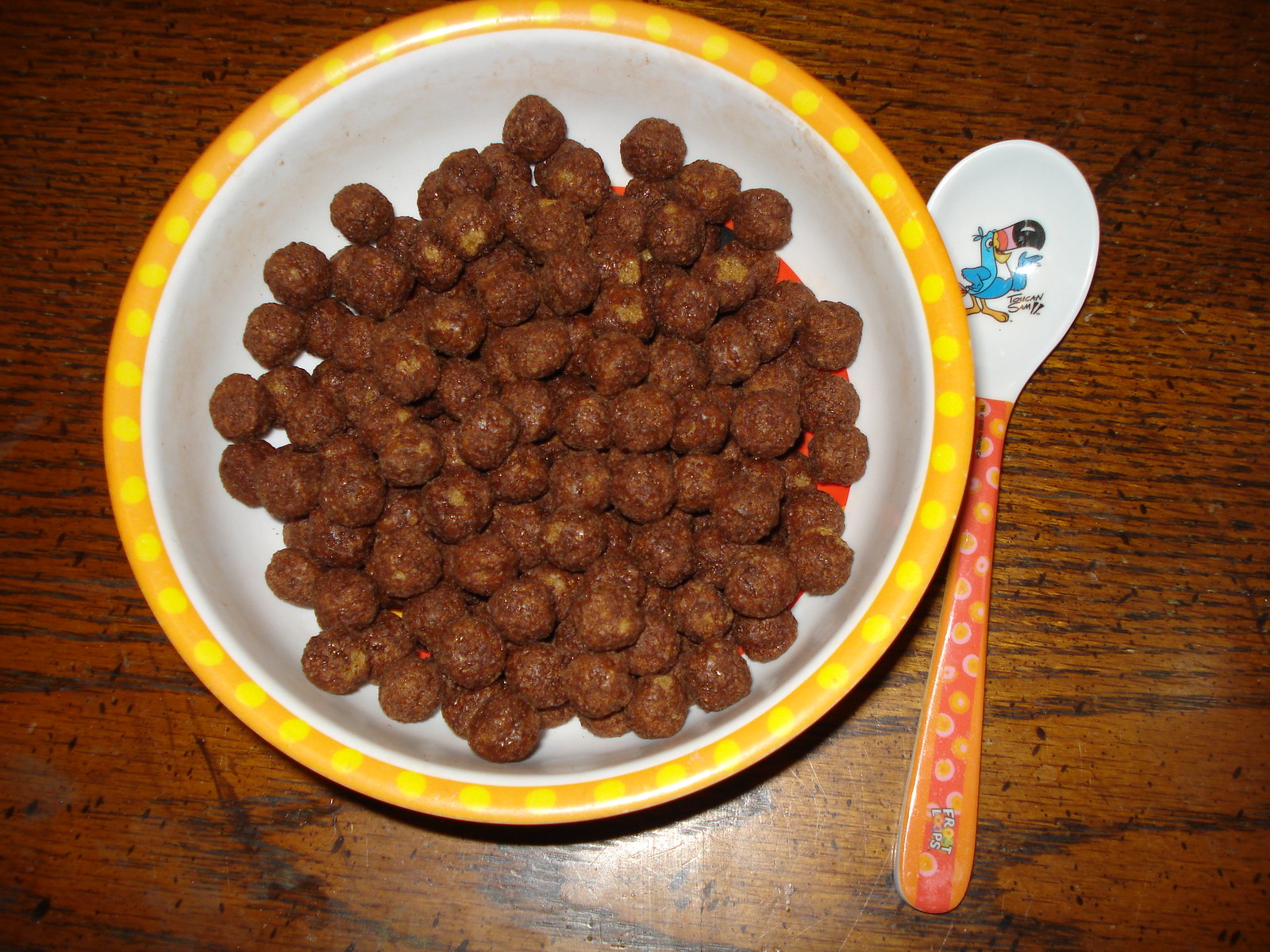The image depicts a child's bowl of cereal placed on a dark brown wooden table with visible wood grain and some signs of wear and tear, such as scuffs and paint marks. The bowl has an orange rim adorned with yellow polka dots and is primarily white inside, though the bottom is obscured by the cereal, which consists of large, round brown puffs resembling Reese's Puffs or another chocolate peanut butter cereal. To the right of the bowl lies a colorful spoon with a red and orange handle featuring circular patterns and the "Froot Loops" logo. The spoon's bowl is white and displays an image of Toucan Sam, a blue toucan with a prominent multicolored beak. Despite the cereal obscuring part of the bowl's interior design, a bit of darker orange peeks through. The overall scene is captured with the use of a camera flash, highlighting the texture and details of the table and breakfast setup.